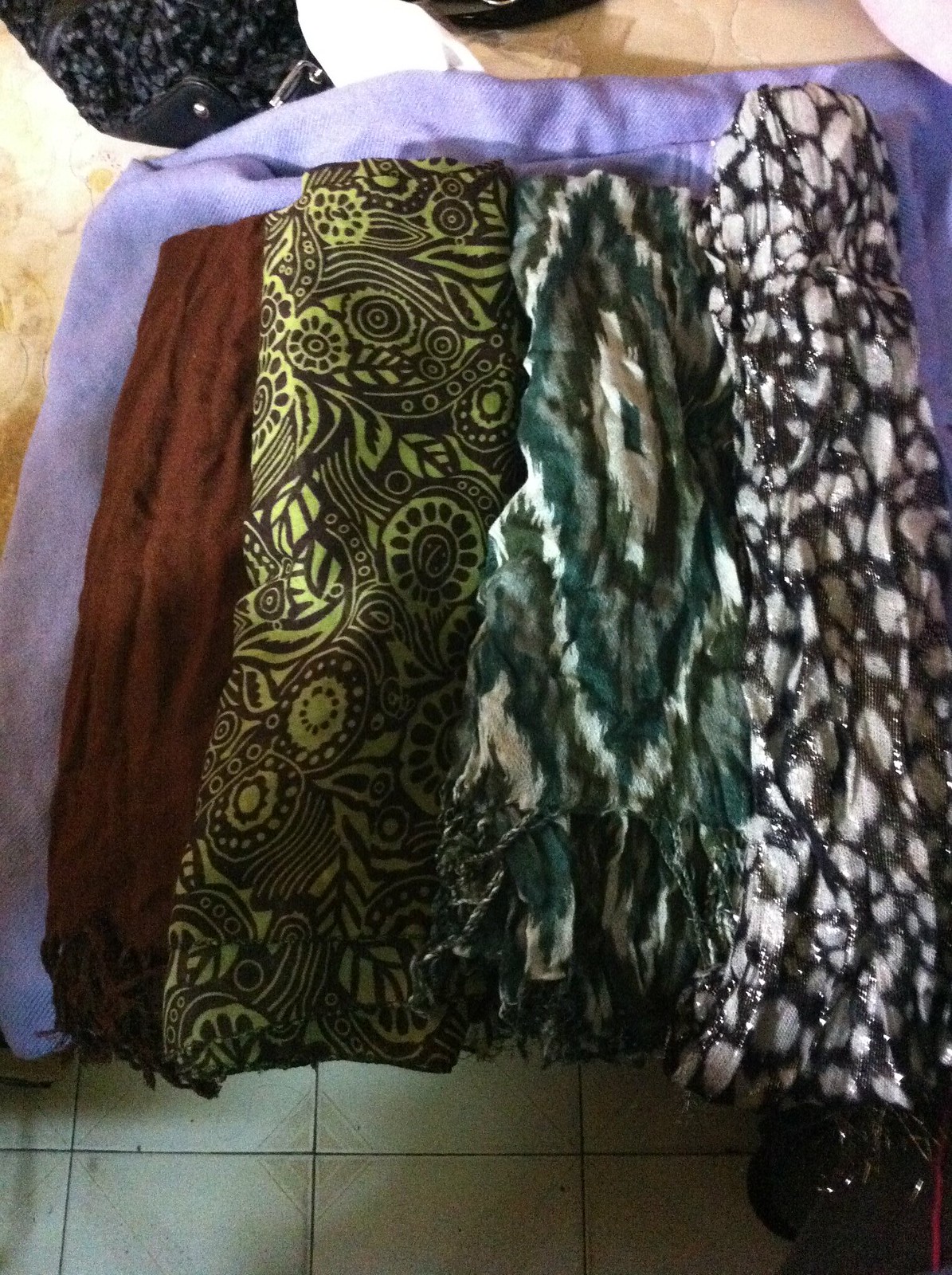The photograph showcases an array of decorative women's scarves meticulously laid out on a fabric-draped surface. The background reveals a bed, with a mattress or comforter visible at the top and a tile floor at the bottom, hinting that the scarves may be cascading over the bed’s edge. The display fabric is blue, serving as a striking base for the diverse collection.

From left to right, the scarves exhibit a variety of colors, patterns, and textures. On the far left, there is a deep maroon scarf. Next, a vibrant red scarf with a fringe at one end. Moving rightward, a yellow and black scarf adorned with floral and leaf motifs sits next to a green and white scarf with a distinctive circular pattern, starting from a green rectangle at the center and expanding outward in green and blue-green rings. 

Further to the right, a dark gray and white scarf characterized by flame-like or feathered designs lies next to a vividly colorful one featuring black and gold accents. A black and white spotted scarf follows, showcasing white dots on a black background. Another patterned piece combines dark green, white, and blue-green hues in a paisley-like arrangement.

On the far right, a white and black scarf with shiny bead-like adornments in the black lines completes the ensemble. This scarf mirrors the meticulous attention to detail seen throughout the entire collection, each scarf adding its unique flair to the cohesive display.